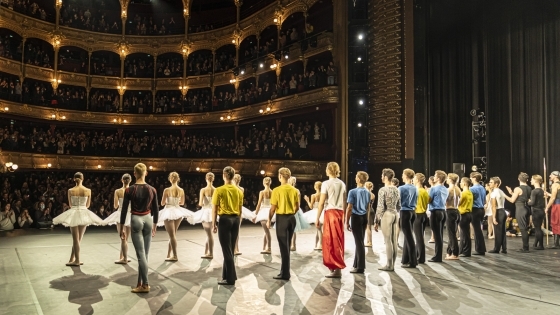The image captures a climactic moment in a large indoor auditorium or concert hall, viewed from the stage. The expansive venue features about four to five levels of balconies, dimly lit except for some scattered individual lights. The audience, filling nearly every seat, is standing and applauding, creating a vibrant atmosphere. On stage, approximately 75 to 100 people are arranged in lines. In the foreground, a line of ballerinas with pointed toes and tutus stand gracefully, their hair neatly pulled back. Behind them are male dancers in fitted leotards or tight pants, some sporting yellow, blue, and white t-shirts, along with potential stagehands in blue shirts and black pants. The entire ensemble faces the audience, reciprocating the applause, celebrating their performance in a grand theater setting.